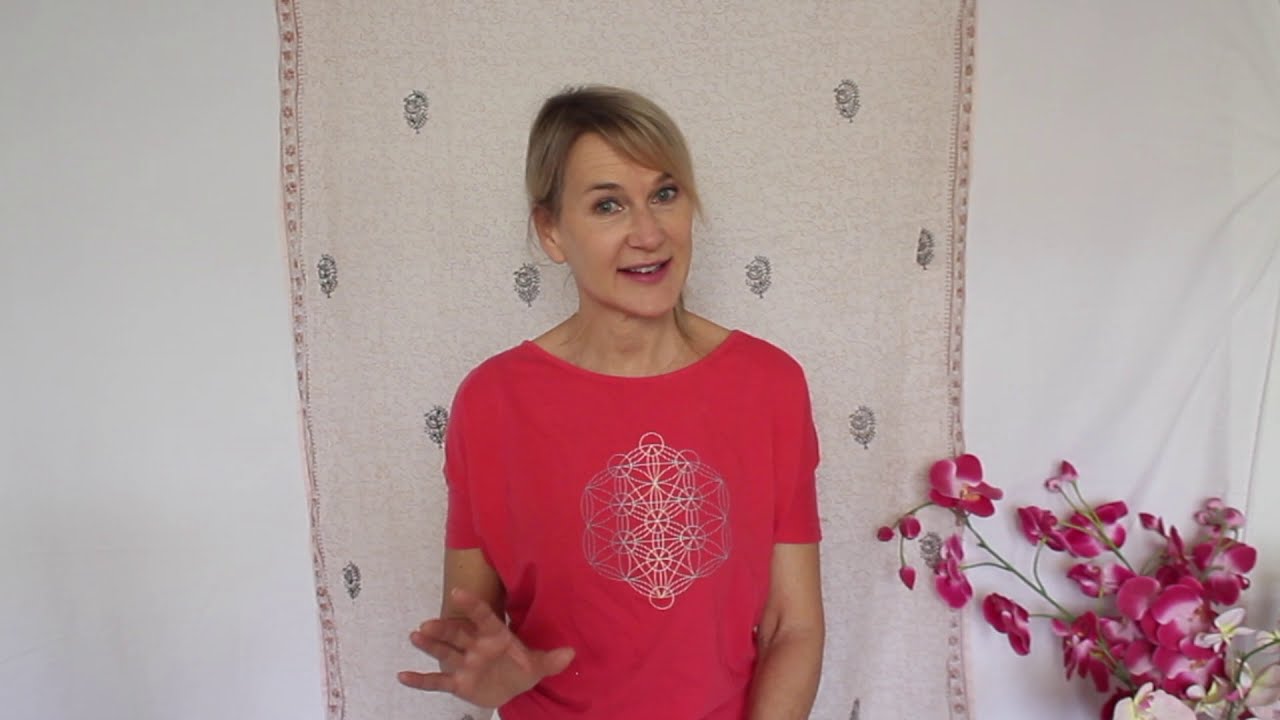The image features a Caucasian woman with dirty blonde hair, dark roots, and at least shoulder-length hair, standing against a white wall with a draped fabric backdrop. The backdrop is a beige or cream-colored curtain adorned with small black flowers, punctuated by a trim of red dots. The woman has hazel eyes and her head is tilted slightly to the right, with her mouth open displaying her upper teeth in a semi-smile. She wears a red, short-sleeved t-shirt with a scoop neck, styled with a geometric design made of interconnected circles. She is gesturing with her left hand raised in a stopping motion, while her right hand hangs by her side. The setting is further decorated with a vase of flowers on the bottom right, containing predominantly red flowers along with smaller white blooms.